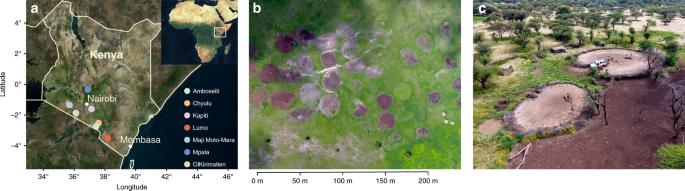The image is composed of three sections laid out as a strip collage, each offering a progressively closer view. On the left (labeled A), is an overhead topographical map of Kenya with an outline of the country, including latitude and longitude markers. The map prominently labels and pins the cities of Mombasa and Nairobi, along with points of interest indicated by the illegible legend. In the center (labeled B), there's a closer aerial view of the Kenyan landscape, presenting a mix of green grassland with circular brown, white, and gray patches, possibly representing natural formations or cleared areas. This photo also includes a scale key at the bottom, measuring up to 200 meters. The image on the right (labeled C) provides an even closer aerial perspective, revealing the brown patches as round, crater-like dirt areas devoid of vegetation, highlighting the detailed texture and possible soil erosion or man-made platforms.